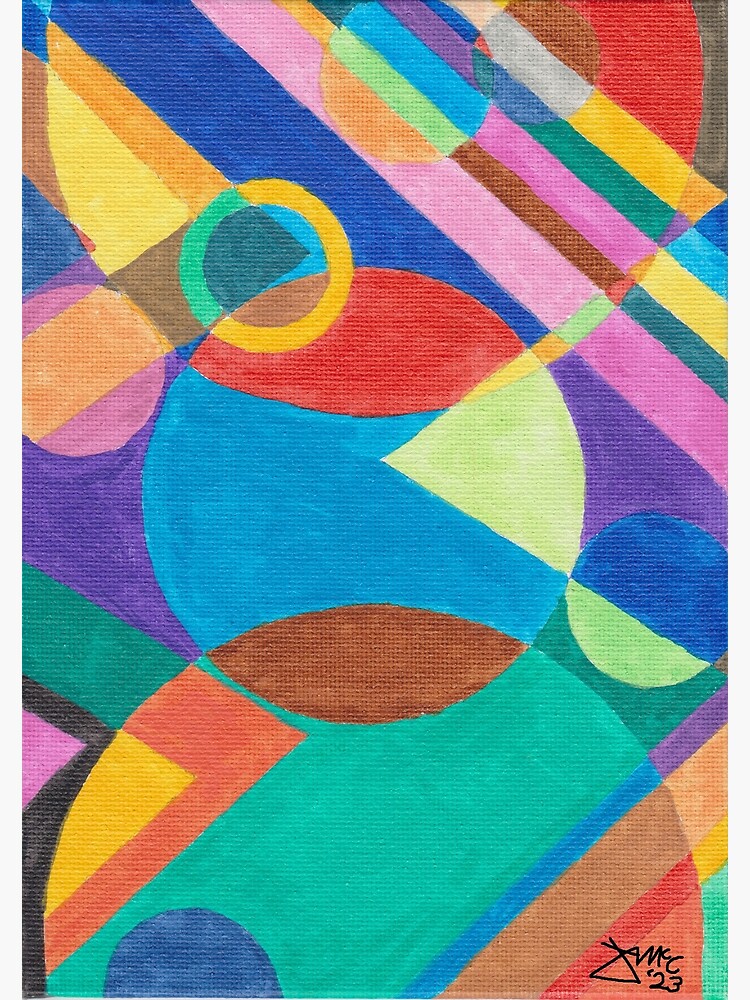The image depicts a vibrant and striking canvas art piece characterized by its colorful geometric shapes. The painting prominently features an array of circles, triangles, arcs, lines, and angles that interweave and overlap, creating new shades and patterns where the colors mix, often in unexpected combinations. The color palette is exuberant and lively, with green, blue, purple, pink, red, yellow, coral, peach, gray, and neon green hues contributing to its dynamic feel, evoking a distinctly 80s aesthetic. Additionally, there is some black in the lower-left section of the artwork. The piece exudes a sense of randomness and creativity, with around ten primary circles and various other shapes intricately arranged. The painting's signature, located in the bottom right-hand corner, reads J.M.C.C. and is dated 2023, marking it as a contemporary work.